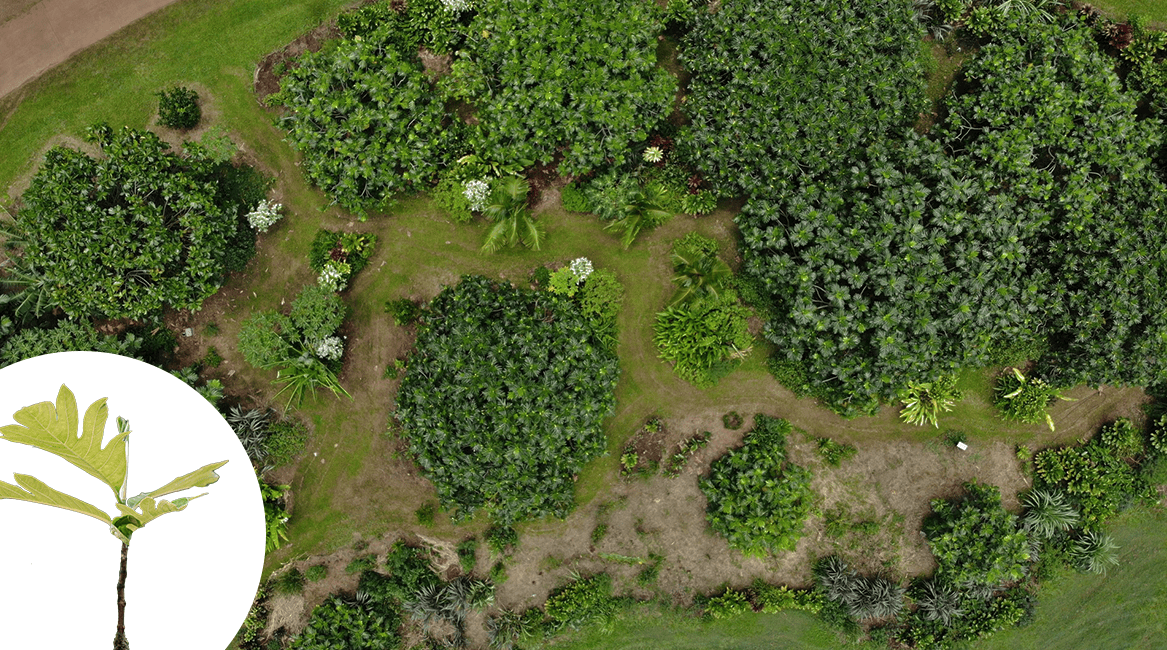This aerial photo, likely taken from a drone about a hundred feet above, shows a meticulously landscaped backyard garden adorned with various plants and pathways. Prominently featured in the top left corner is a medium-sized green shrub adorned with white flowers, surrounded by other similarly sized shrubs. Interspersed between these larger plants are smaller plants with white blossoms that appear as singular flowers due to their clustered arrangement. On the lower right side, there are plants with vibrant yellow flowers. The garden is segmented by winding pathways and bordered on one side by a sidewalk, creating an organized structure amidst the lush vegetation. The diverse flora includes round-shaped trees and bushes, patches of ferns, and several shrubs with white blossoms. The garden's greenery exhibits a range of shades, from darker, deep greens to lighter, brighter hues. Additionally, there are sections of bare dirt and grassy areas. A distinctive feature in the lower left corner is a half-circular arrangement with a notable plant standing in its center, contributing to the garden's varied and picturesque landscape.